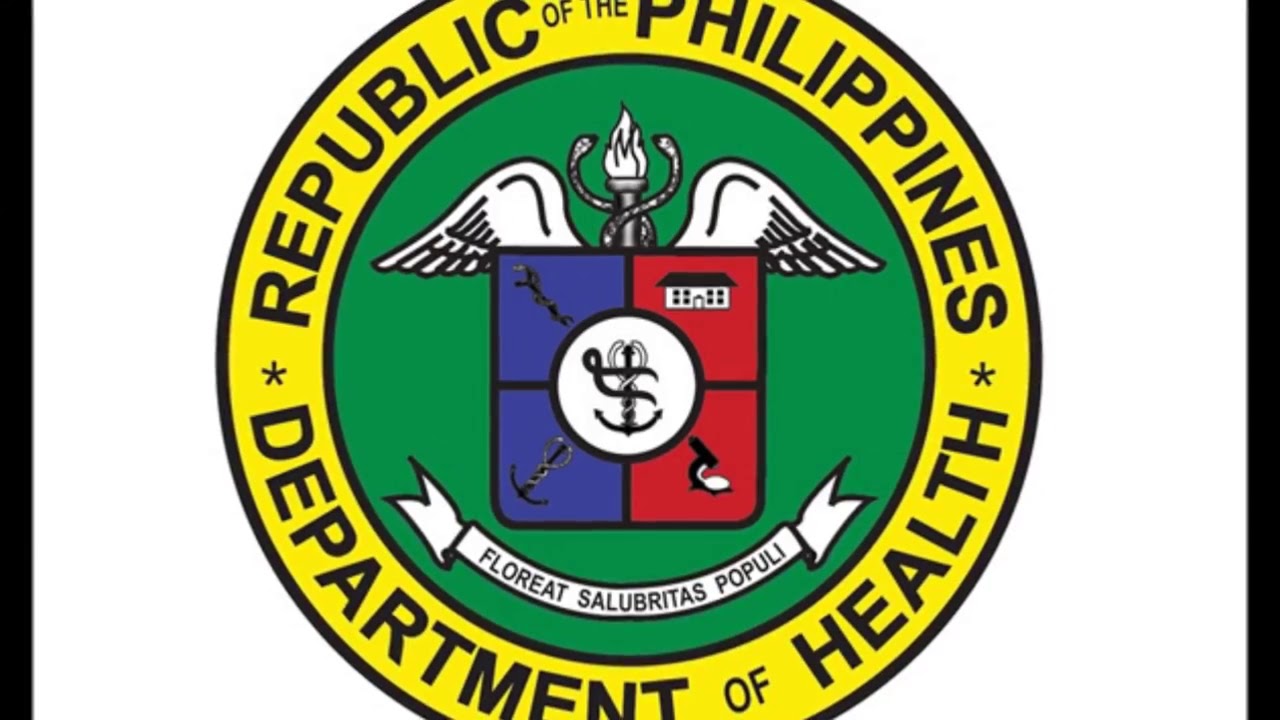The image is a horizontally aligned rectangular emblem with thick black borders on the left and right sides, framing a white background. In the center of this background is a prominent circular seal, bordered by a black outline. Encircling the edges of this seal is a yellow ring with the inscription "Republic of the Philippines" at the top and "Department of Health" at the bottom. Within this yellow ring is an inner green circle, also bordered by a black outline.

At the heart of the green circle lies a square divided into four quadrants, each containing distinct imagery: the top left quadrant seems to depict an anchor, the top right a house, the bottom left a wrench, and the bottom right a shoe. At the top of this square is an intricate design featuring wings, a flame, and two coiling snakes. Below the square is a white banner inscribed with the Latin phrase "Floreat Salubritas Populi," meaning "Let the Health of the People Flourish." The rest of the seal and the surrounding image retain a clean white background, emphasizing the elements of the emblem.